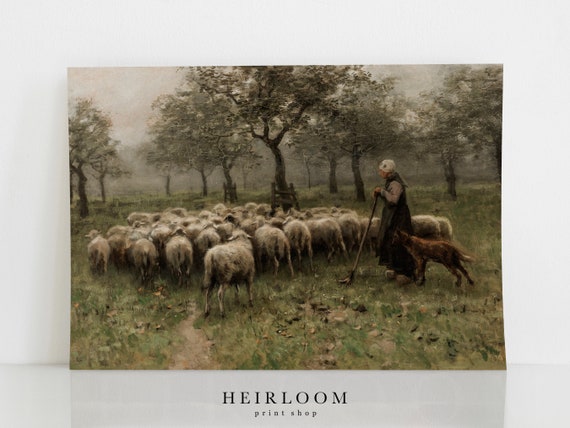The framed artwork, labeled "HEIRLOOM" in capital letters and "print shop" in lowercase beneath, depicts a serene outdoor scene. In the foreground, a person wearing a dark robe and form-fitting white hat stands on the right side, holding a long pole—likely a shepherd. Positioned beside them is a brown dog, attentive and poised. Central to the image, a large herd of about 30 to 40 sheep, primarily grayish in color, are clustered together, many bent over grazing in the field. Behind this pastoral group, trees dot the background, enhancing the tranquil rural setting. The entire scene is set against the backdrop of a white museum-like wall, indicating its display as a piece of art.